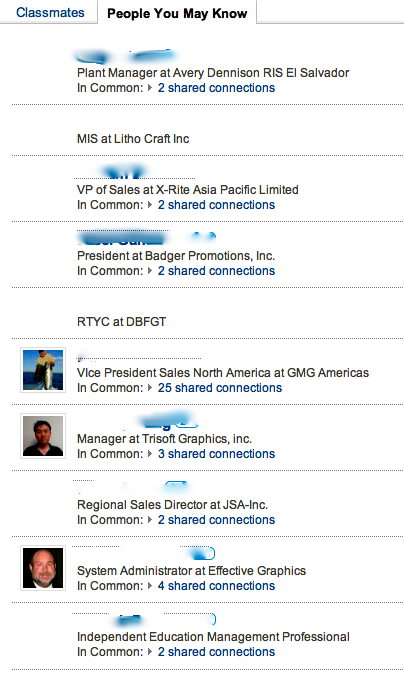The image depicts a vertical rectangular page with a white background. At the very top left, there is a white button displaying the word "classmates" in bright blue text. To its right, in black text, it reads "people you may know." Below this heading is a vertical list of people. 

Each entry starts with a person's name and photo, both of which are either blacked out or grayed out. The first entry beneath the heading has a gray text description: "Plant Manager at Avery Dennison, RIS, El Salvador." Following this, it reads "2 shared connections" in bright blue text. 

The second entry also has the person's name and photo blurred out, and their position is listed as "VP of Sales at Xrite Asia Pacific Limited" in gray text. Again, "2 shared connections" appears in bright blue text. 

The third entry—continuing the format—has an omitted name but includes a photograph in a square on the left. The position is described in gray text as "Vice President Sales North America at GMG Americas." The line below states "25 shared connections," with the shared connections number highlighted in bright blue text. 

These profiles extend further down the page, maintaining the pattern of omitted names while some connections have available photos. The connections cover different professional titles and shared connections among the users.